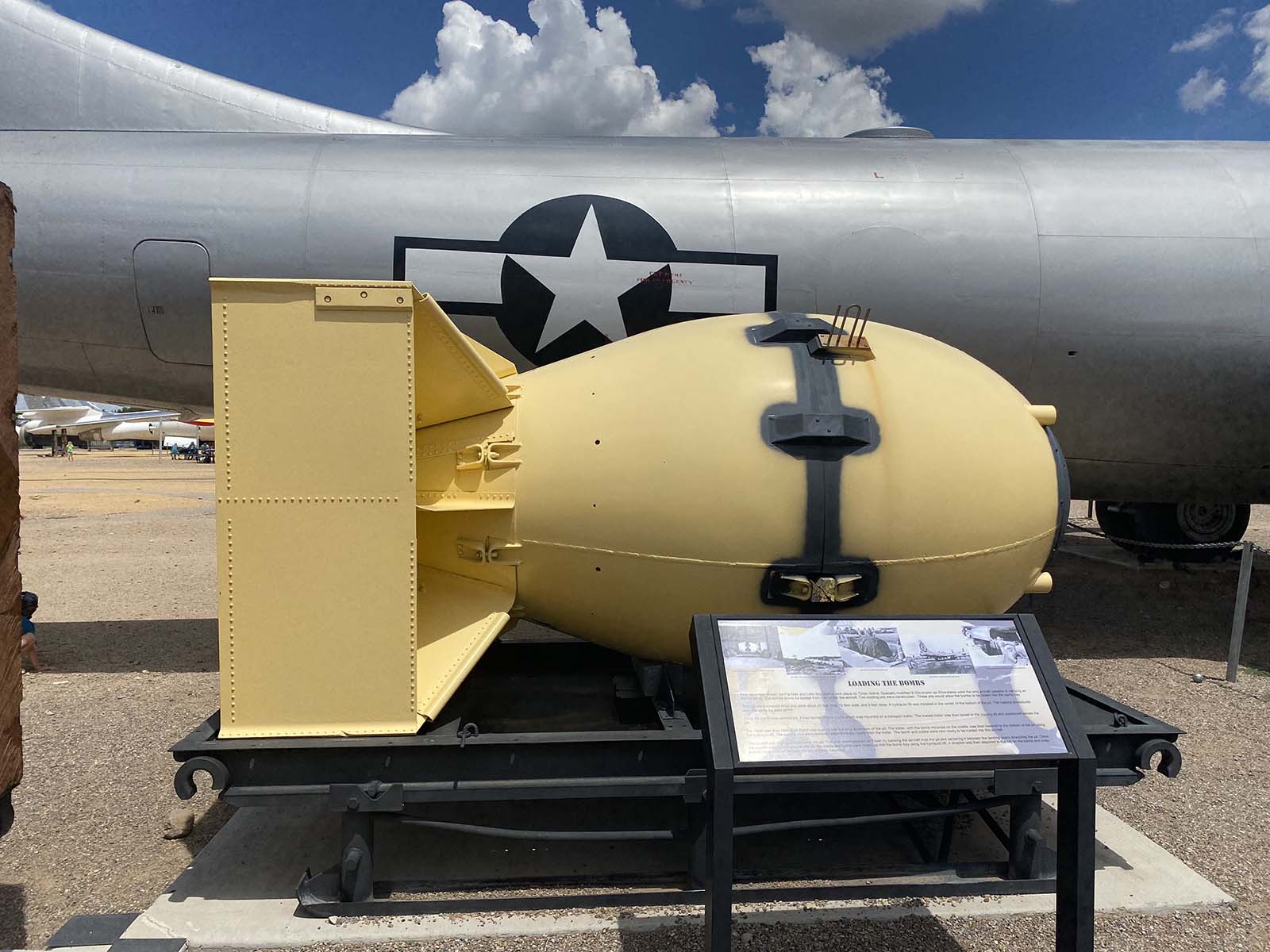This daytime photograph, likely taken at an air show or airplane museum, features a backdrop of a clear blue sky with scattered clouds. The focus of the image is a cylindrical, beige-colored device adorned with a gray band. This device, resembling a bomb casing or a grenade, rests on a gray metal platform. In front of it, a plaque provides detailed information about the device, including its usage and history.

Prominently featured behind the device is a large gray airplane, which bears an emblem consisting of a blue circle with a silver star in the center. The setting appears to be a concrete area, possibly a tarmac, and additional planes can be seen in the background underneath the main aircraft. The scene captures a historical exhibit of military aviation equipment under a sunny sky, reflecting the heritage of air combat technology.